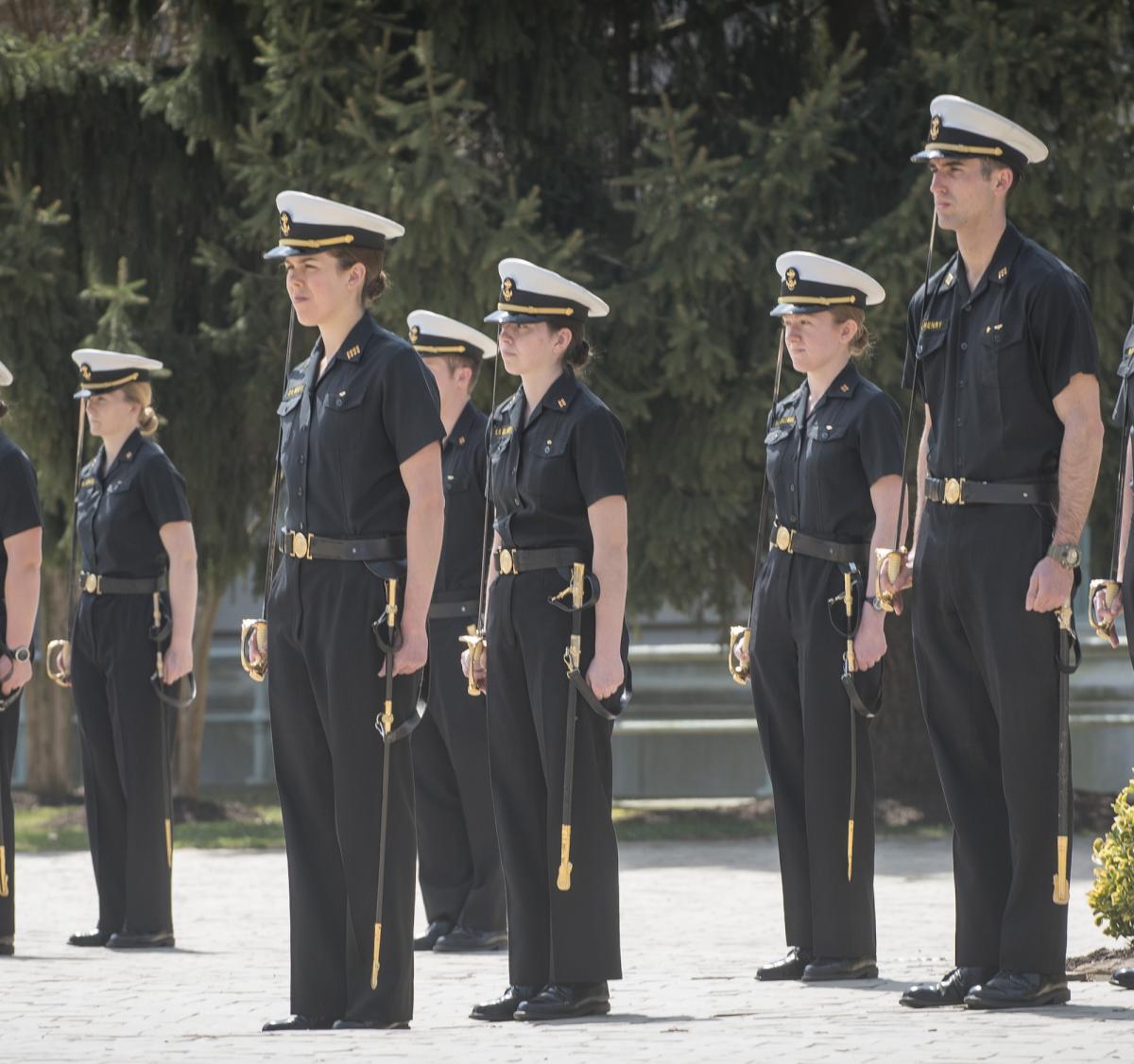The photograph captures seven service members, positioned in two rows, standing at ease with their weapons—likely swords—held on their shoulders. All are dressed in either dark navy or black uniforms, complemented by white hats with black brims and gold cords above the visors, which bear the symbol of an anchor. Their attire is further detailed with gold buttons and black belts featuring gold clips. A scabbard can be observed on each member's hip. The service members maintain a reserved and neutral expression, looking straight ahead. Behind them, a large pine tree and some grass and trees add to the backdrop, along with a partially visible building at the bottom of the scene. The soldiers' appearance is uniform, right down to their polished black shoes. One member is noticeably cut off by the edge of the photograph, although their watch remains visible. The image focuses on the disciplined stance and detailed attire of the military personnel, likely from a branch of the Navy, in a moment of poised readiness.